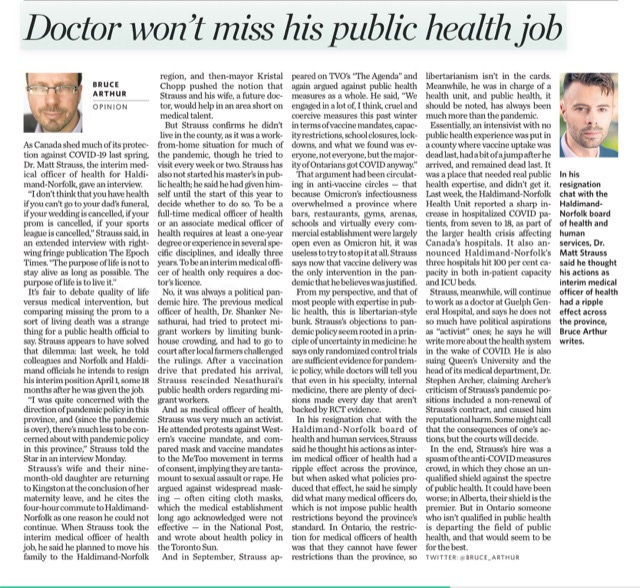At the top of the image, there's a pale greenish-gray box with black text reading, "Doctor Won't Miss His Public Health Job." The article's author, Bruce Arthur, is also mentioned. It is an opinion piece and features two images: the first one is of a bespectacled man with slight facial stubble, identified as Dr. Matt Strauss, and the second image shows a brown-haired man without glasses, dressed in a suit.

The article discusses how Canada relaxed many of its COVID-19 protections last spring. Dr. Matt Strauss, Interim Medical Officer of Health for Haldimand-Norfolk, gave an interview where he stated, "I don't think that you have health if you don't go to your dad's funeral, if your wedding is canceled, if your prom is canceled, if your sports league is canceled." He further elaborated in an interview with the right-wing publication Epoch Times, saying, "The purpose of life is not to stay alive as long as possible; the purpose of life is to live it."

Such statements sparked debate over the quality of life versus medical intervention, and Strauss's comments, comparing missing significant life events to a 'sort of living death,' were particularly controversial coming from a public health official. Last week, Strauss indicated he would resign from his interim position on April 1st, approximately 18 months after assuming the role, citing commuting issues and the conclusion of his wife's maternity leave as factors.

Strauss originally intended to move his family to the Haldimand-Norfolk region but did not follow through and largely worked from home. His tenure was marked by a notable shift from his predecessor, Dr. Shanker Nesathurai, who had implemented strict measures to protect migrant workers. Strauss rescinded many of Nesathurai's public health orders and became a vocal activist against many pandemic mandates, including vaccines and mask requirements, often publicly aligning himself with libertarian views.

The controversy surrounding Strauss is further fueled by his public statements and writings, arguing against widespread masking and vaccine mandates, comparing them to coercive measures. Despite these contentious views, Strauss mentioned that vaccine delivery was the only justified intervention during the pandemic.

Underneath the article, the second image's caption states that in his resignation chat with the Haldimand-Norfolk Board of Health and Social Services, Dr. Matt Strauss believed his actions as Interim Medical Officer of Health had a significant impact across the province, as noted by Bruce Arthur.